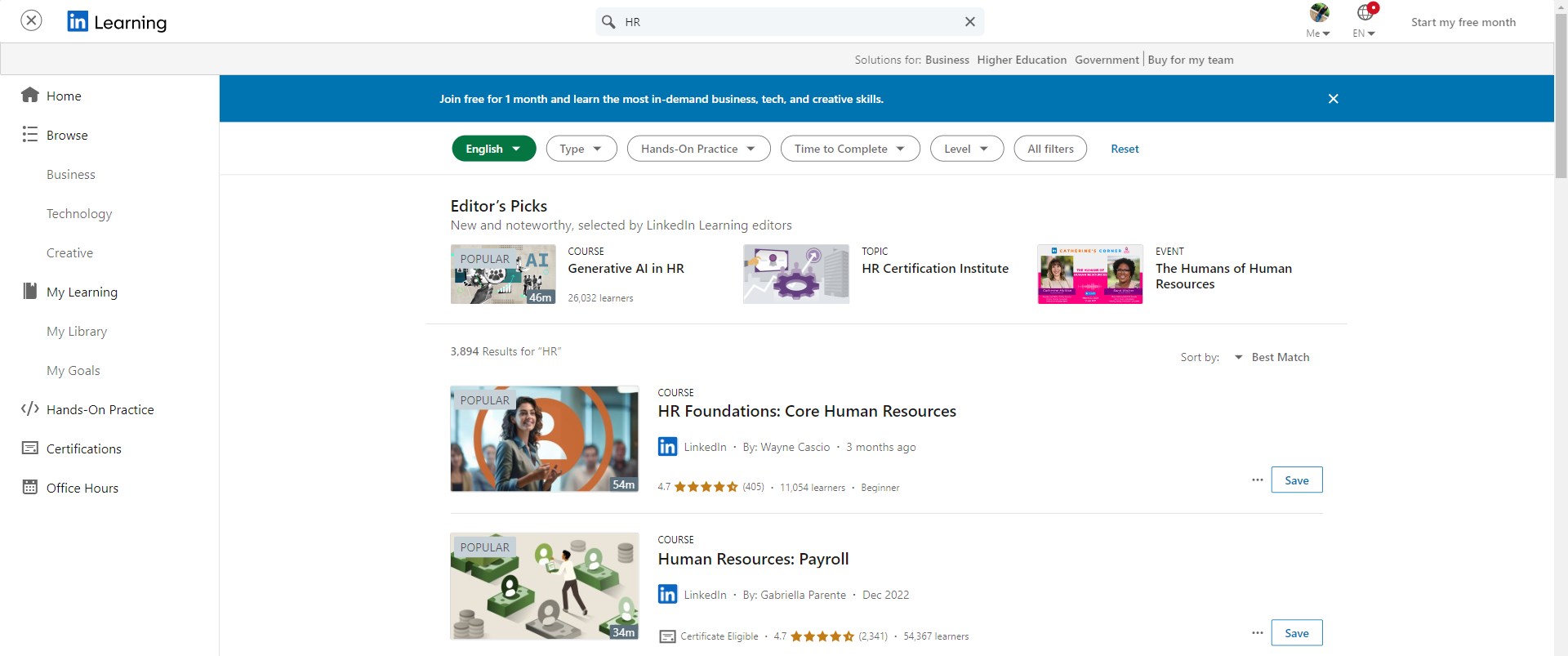### Descriptive Caption for Navigation Menu Image

At the very top of the image, there's a small blue square containing the letters "I-N," adjacent to the word "Learning." Beneath this section, there are options organized vertically: "Home," "Business," "Technology," "Creative," followed by a folder icon linked to "My Learning," "My Library," "My Goals," "Hands-On Practice," "Certification," and "Office Hours."

Moving to the right side of the image, the heading "Editor's Picks" is prominently displayed. Below this, there's a section titled "Generative AI," presented within a square frame. Adjacent to this square is another box showcasing a purple settings wheel icon, labeled "HR Certification."

Further to the right is a feature titled "Humans of Human Resources," displaying two images of different women against a pink background. Below this is a segment for the course "HR Foundations: Core Human Resources," which includes an image of a woman standing in an office setting.

Beneath this section are multiple green squares, each containing a white icon of a person in profile, representing "Human Resources Payroll Course." The upper left corner of this square has the label "Popular." In the upper right corner of the image, a small red circle is present next to the text "Start My Results."